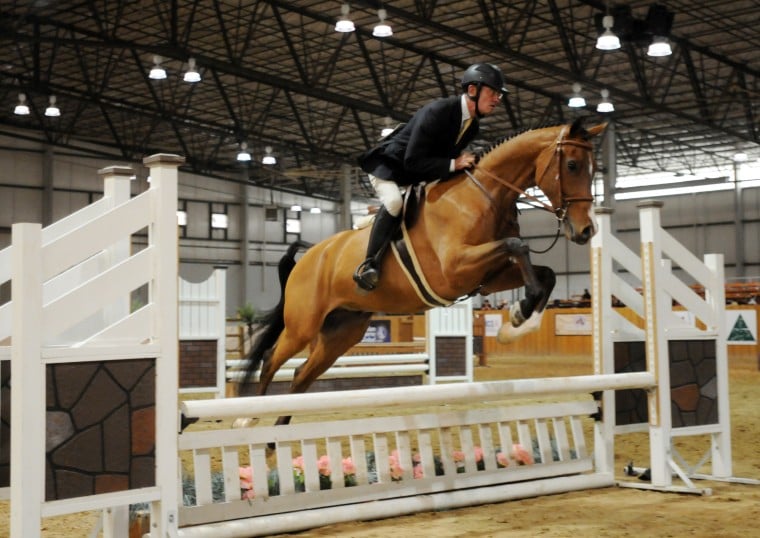Inside a spacious equestrian practice arena, a skilled horse rider is captured in action. The high ceiling, adorned with hanging lights, illuminates the indoor space, while distant audience seats suggest a venue designed for both practice and competition. The rider, dressed in traditional equestrian attire including a helmet and long black boots, exhibits poise and concentration. Mounted on a light brown horse, the pair is mid-leap over a white gate, showcasing both the athleticism of the horse and the expertise of the rider in this dynamic moment.